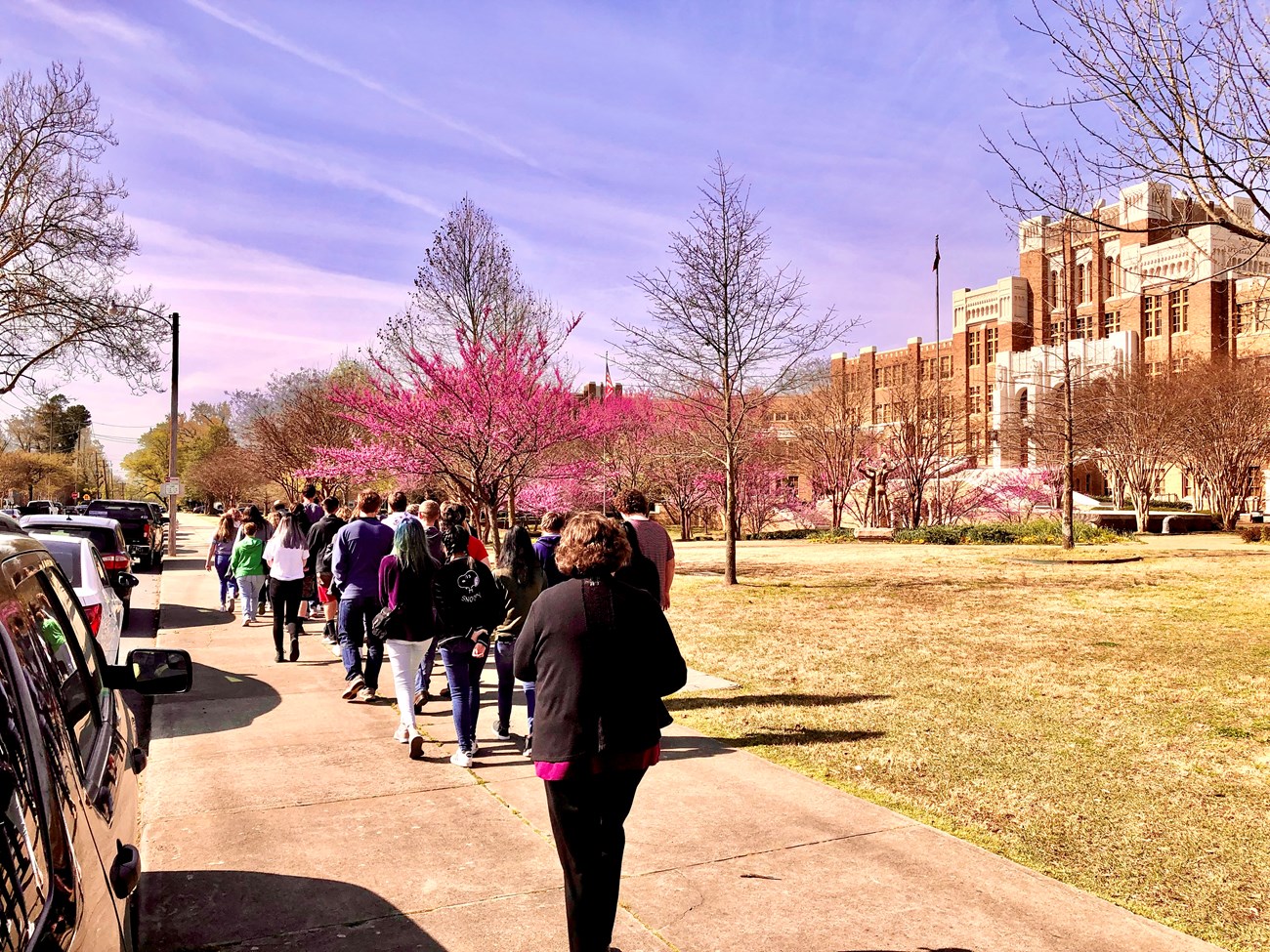In this color photo taken during a clear, blue-skied day with white cirrus clouds, a group of approximately 20 people walk along a sidewalk with their backs turned. They are dressed in pants and jackets, suggestive of cooler weather, possibly fall. To their left, a line of cars is parked along the curb, while to their right, there is a large red brick university building adorned with white or tan accents. Before the building, there is a spacious, mowed lawn that appears mostly dead, showing yellow and brown grass. The landscape includes a mix of bare trees and some with pink or purple flowers, contributing to the autumnal atmosphere of the scene.